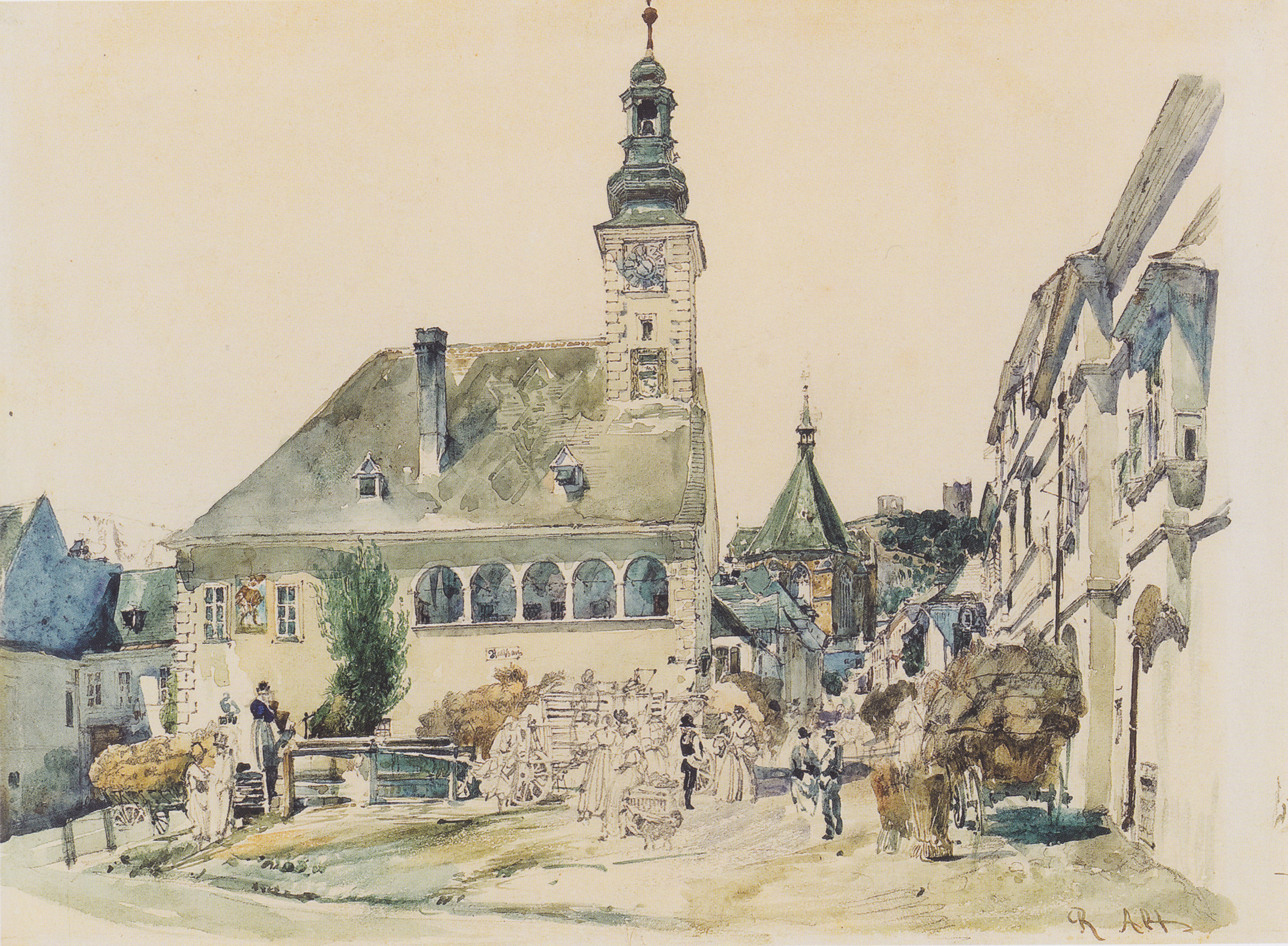This watercolor painting, signed in the bottom right-hand corner with an "R" followed by what appears to be "A, P, T" or "ATS," depicts an old-fashioned European town, likely from the 16th to 18th centuries. The scene is imbued with soft, subtle tones and neutral colors, predominantly pale white, off-white, beige, with hints of tan and light olive green. The background is an expansive, overcast gray sky, which sets a muted atmosphere.

In the foreground stands an imposing Victorian-era building with a tall bell tower or spire, topped with a weather vane instead of a cross, suggesting it might be an official building rather than a church. The tower roof is an off-green shade, and the building features domed windows reminiscent of stained glass. Surrounding this main structure, the attire of the figures—black suits and long dresses—suggests a 19th-century setting, though individual facial features are deliberately vague, contributing to a sketch-like quality.

The street scene is bustling with activity: two men chat in front of the building, a woman appears to be working on the side of a house, and others stroll about. A dog waits expectantly near a table that looks like a makeshift stall displaying goods. Various wagons, one filled with straw, and a cart are scattered around, indicating a market or communal gathering place. The right-hand side of the painting features continuous rows of buildings that might be houses or apartments, showing windows and doorways but little of their roofs.

Overall, this painting rich in historical ambiance and subtle details provides a nostalgic glimpse into a European town's streetscape from centuries past, capturing the charm and simplicity of daily life in a bygone era.